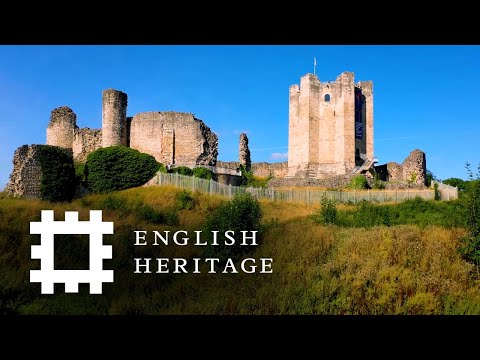This image features the ruins of a medieval castle, characterized by its deteriorated walls and structures. Prominently on the left side, two moderately intact towers rise above the crumbling wall. The castle's interior backdrop reveals a large, dilapidated building and several almost completely deteriorated towers. A white security fence encircles this historical structure, indicating efforts to preserve it. In the foreground, a significant black and gray rock formation, showing signs of wear, sits alongside dense shrubs, weeds, and varied yellowish-green grass.

The sky is a bright blue, dotted with a few white clouds, enhancing the serene yet poignant atmosphere of the scene. In the bottom left corner of the image, a white square with hatch marks adjacent to the text "English Heritage" suggests the location is maintained by this organization. The image is framed by thick black borders at the top and bottom, giving it an official, perhaps promotional appearance.